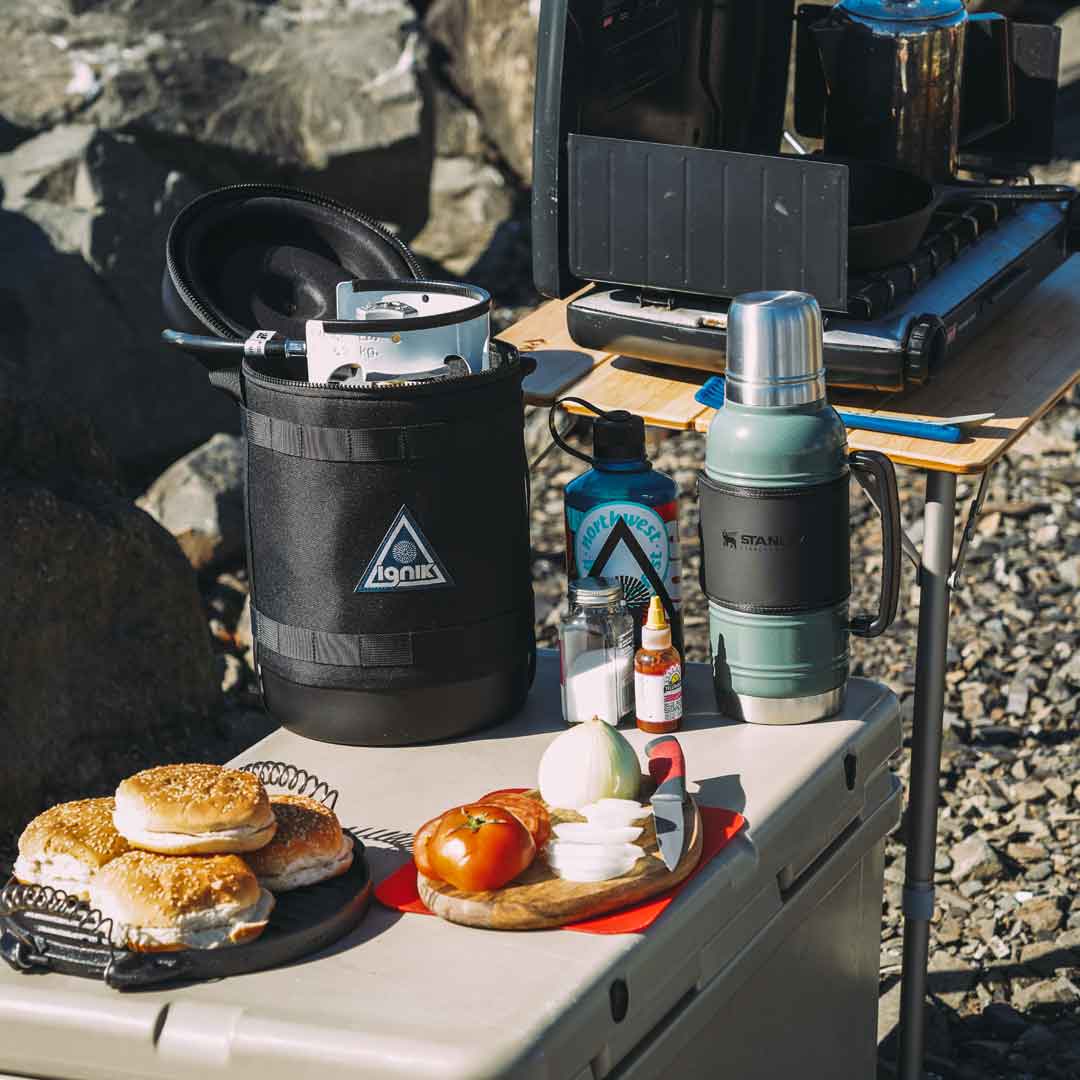This outdoor scene shows a detailed campsite setup where people are preparing a meal. The ground is covered with gravel and larger rocks, and the sun is shining brightly. A white cooler serves as the foreground focal point, topped with an array of food preparation items. A black dish holds hamburger buns with white seeds, and next to it, a red plate supports a brown cutting board with sliced tomatoes, a whole white onion, and onion slices. A sharp knife with a red and black handle lies on the board. Nearby, there is a clear bottle of white powder, a red bottle of hot sauce, and a Coleman Stanley thermos. Also in view is a black padded container holding a white propane canister labeled "IGNIK." Behind the cooler, a wooden table displays a large Coleman stove, and an adjacent folding table supports additional cooking equipment, including a cast-iron skillet. The overall atmosphere conveys a well-organized outdoor cooking area, ready for barbecue or lunch preparation.